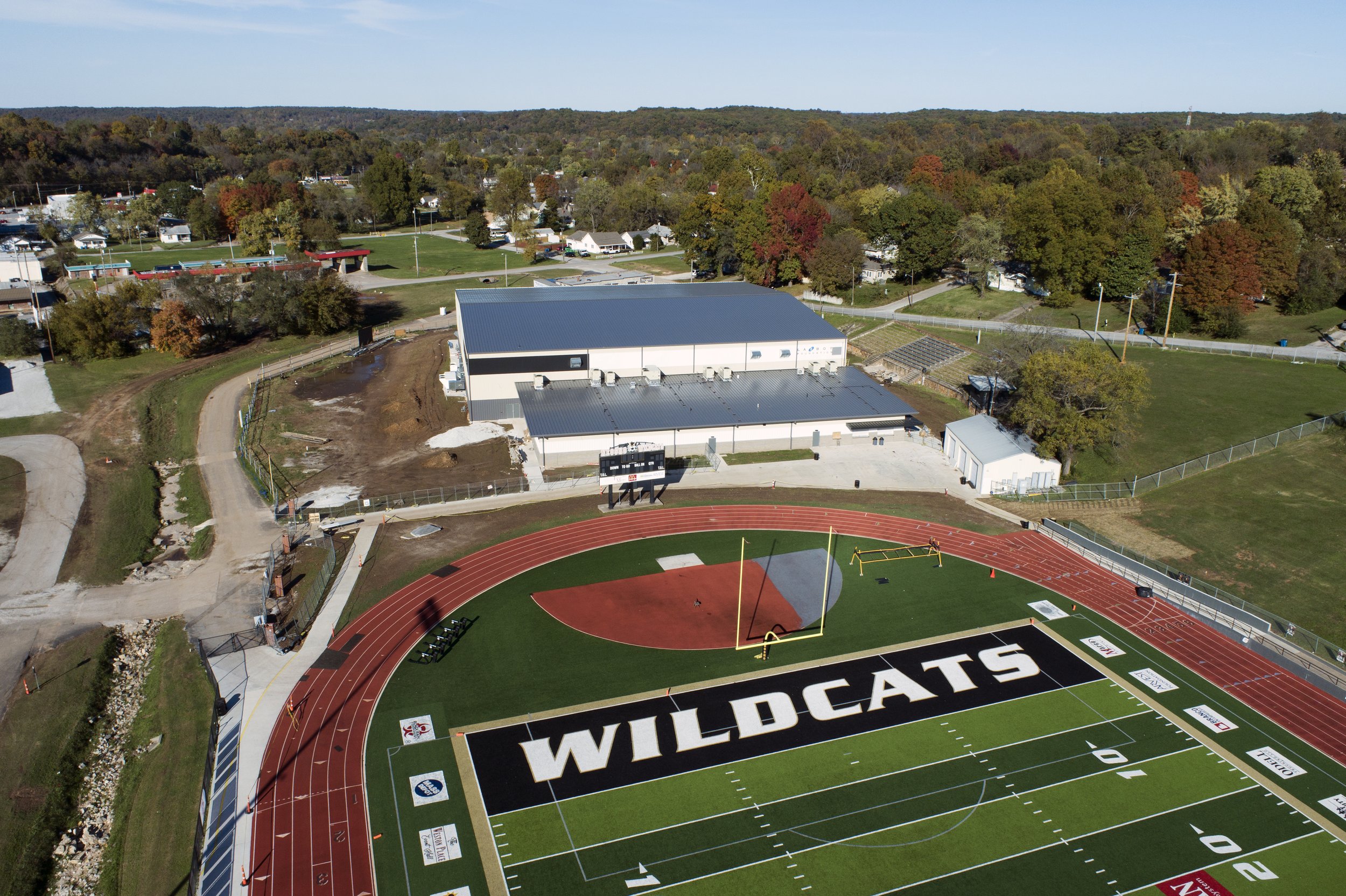This detailed aerial photograph captures a vibrant, multi-layered scene centered around a football stadium. At the forefront of the image, prominently situated in the middle-right, is a well-maintained football field, where "Wildcats" is visibly emblazoned in white on a black end zone. Surrounding the field is a red, or reddish-orange running track, clear and unmistakable.

Encircling the stadium are two white buildings with distinct gray, slate gunmetal roofs; one larger and one smaller, possibly suggesting a field house or gymnasium that connects to the main structure. Stadium seating is visible, indicating well-planned viewing areas for spectators.

Beyond the immediate vicinity of the stadium, the photograph reveals a broader landscape. A network of roads and houses populate the mid-ground, indicating a nearby town or residential area. Dominating the upper portion of the image are dense patches of green and red trees, suggesting a forest with a mix of deciduous trees transitioning through autumn colors. Above this verdant expanse, the sky stretches across the top border of the image, painted in a light blue hue with a scattering of white clouds primarily on the left side.

Additional details include the alternating dark and light green stripes marking the football field, clear demarcations of the 10-yard and 20-yard lines, and a few people captured mid-activity on the track, adding a lively element to the composition. This aerial photograph masterfully encapsulates a bustling, diverse environment centered around an active football stadium, framed by natural and residential landscapes.